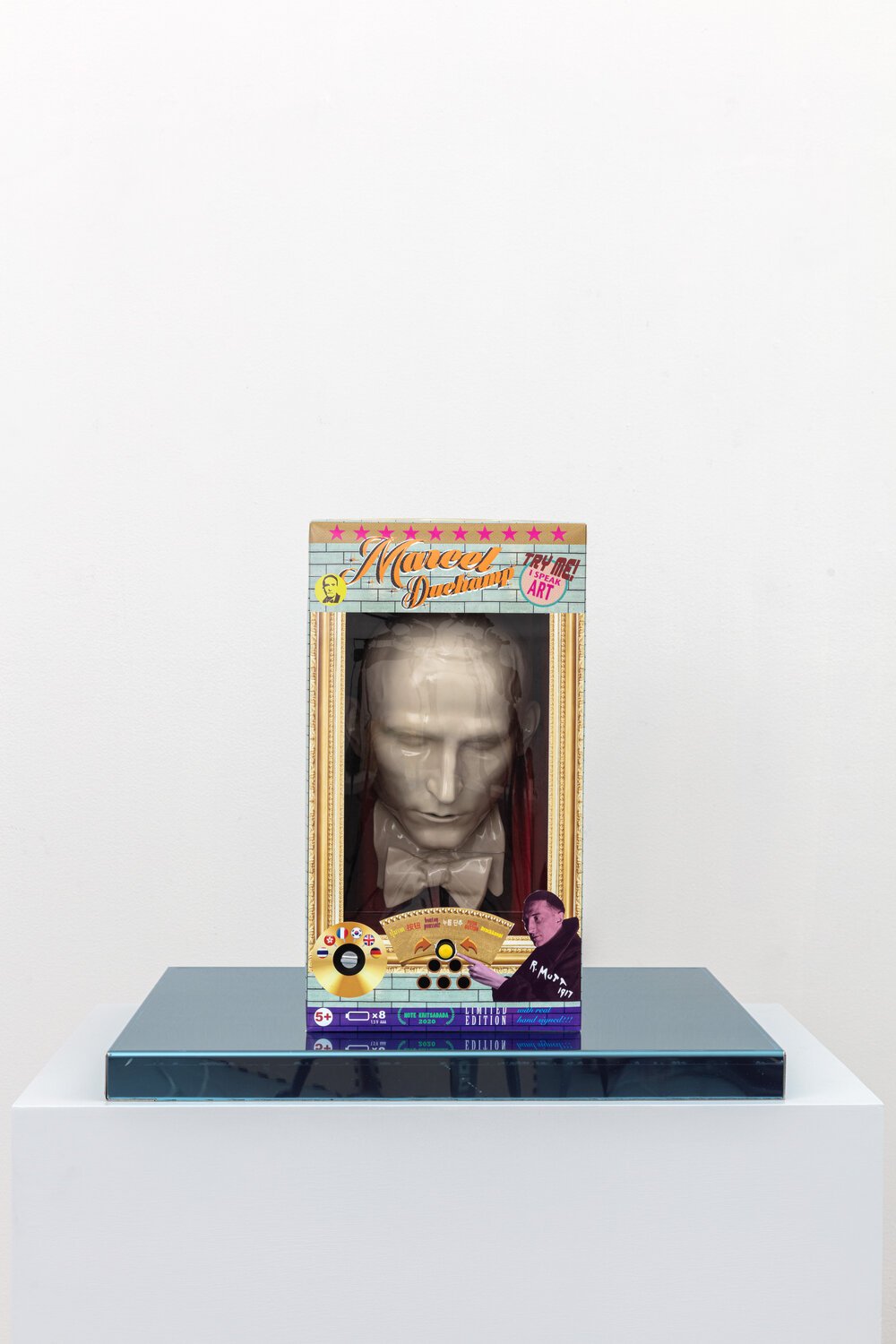The image depicts a limited edition collectible figure of Marcel Duchamp. The background is predominantly white, providing a clean and unobtrusive backdrop. At the bottom of the image is a white rectangular box acting as a pedestal. On top of this pedestal sits a striking aquamarine, bright blue metallic rectangular surface, which is reflective and approximately an inch thick, positioned to form a table. Resting atop this blue surface is the main collectible: a cardboard box with a plastic window showcasing a head sculpture of Marcel Duchamp. The box features rich detailing, including a purple base that transitions into a gray stripe, and is adorned with gold gilded picture frames on each side. The top of the box presents a gray brick pattern. Inside, the black-and-white head sculpture of an older man, resembling Marcel Duchamp adorned with a powdered wig and a white bow tie, can be seen. The box is labeled with "Marcel Duchamp" in gray and orange writing and includes a brown bar with multiple hot pink stars. Additional features described include a "Try Me, I Speak Art" label with pink stars, and a yellow button that, when pressed, plays art-related phrases in different languages, adjustable via a side button. The collector's item is presented in a visually striking manner, emphasizing its limited-edition status with intricate design elements and interactive components.